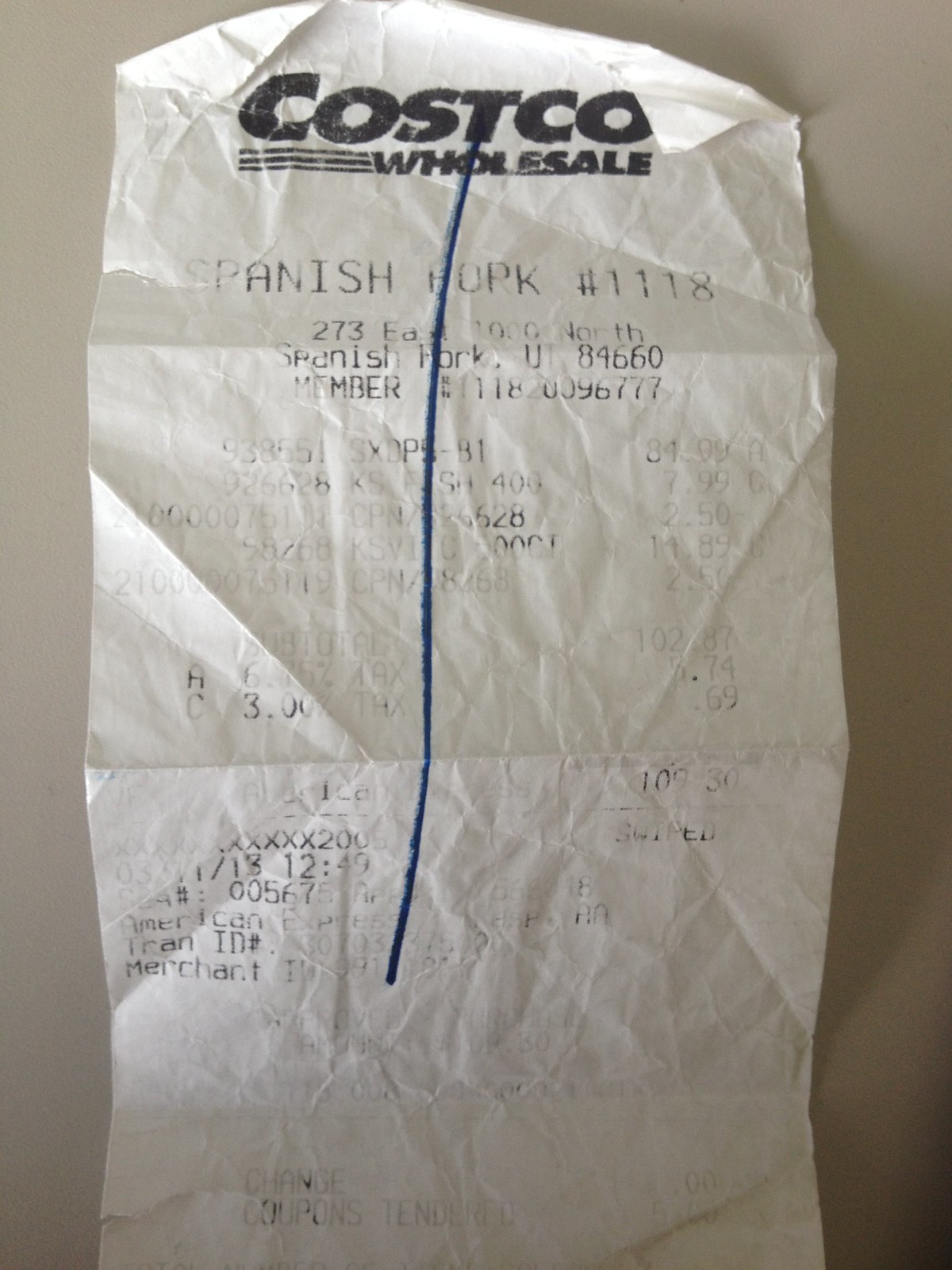A crumpled white receipt lies against a light gray background, showcasing black printed text. The receipt's top two corners are noticeably curled downward. The prominent heading reads "Costco Wholesale" in bold black letters. A pronounced blue pen mark runs vertically down the center of the receipt. While the text is faded and much of it is illegible, the words "Spanish Pork" can be faintly discerned. The purchase time is indicated as being sometime after 12 noon. The paper is heavily wrinkled, adding a textured, worn appearance to the image.